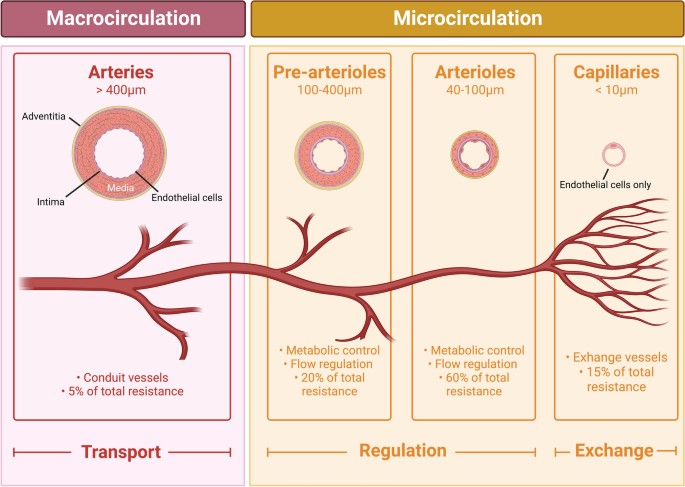The medical diagram is a rectangular flow chart depicting the hierarchy and function of blood vessels, mapping the journey from larger to smaller vessels from left to right. The chart is divided into two main sections highlighted by distinct background colors: a pink section on the left and a yellow section on the right, both titled "Macrocirculation." 

In the pink section on the left, a circular diagram labeled "arteries" greater than 400 µm (micrometers) includes anatomical details such as "adventitia," "intima," "endothelial cells," and "media." This section is also marked as "conduit vessels" with a note stating they account for 5% of total resistance, emphasizing the transport function of these vessels.

The yellow section on the right is divided into three subsections: prearterioles, arterioles, and capillaries, together labeled "Microcirculation." Prearterioles, ranging from 100 to 400 µm, are involved in "metabolic control" and "flow regulation," comprising 20% of total resistance. Arterioles, sized 40 to 100 µm, are also involved in "metabolic control" and "flow regulation," but account for a higher resistance at 60%. The smallest vessels, capillaries, measuring less than 10 µm, are identified as "exchange vessels" dealing solely with "exchange" functions, composed entirely of endothelial cells, and comprising 15% of total resistance.

Throughout the chart, a continuous red depiction of a blood vessel sweeps from left to right, visually linking all sections and highlighting the transition from larger conduit arteries to tiny exchange capillaries.